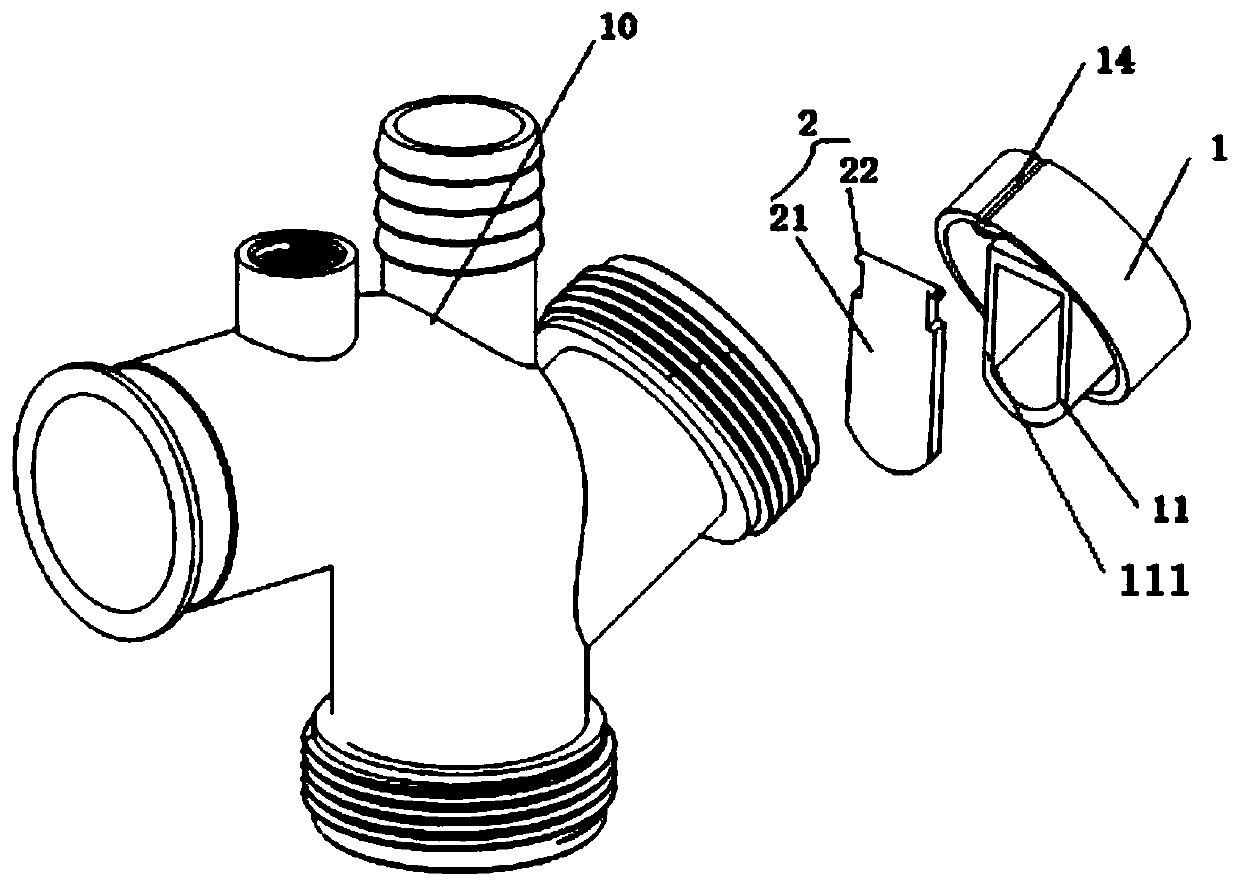The black and white diagram displays a detailed and labeled illustration of a multi-opening pipe fitting against a solid white background. The primary object, outlined in black, features four circular openings: one at the bottom with visible grooves for hose attachment, one spout extending to the left, another hose attachment on the right side, and a final opening at the top. This main structure is marked with the number 10 at the top.

Adjacent to the main object, on the right side, is a secondary piece resembling a flap or shield shape. This piece is labeled with the numbers 2, 21, and 22, indicating different areas of the flap. Further to the right, there is a third circular component, which appears to have a hole designed to fit with the shield-shaped piece. This circular component has several labels: number 1 pointing to its side, number 11 indicating an attachment point, number 111 pointing to another part, and number 14 highlighting a groove on its top. Together, these elements seem to form a comprehensive diagram, possibly related to a hose attachment or a plumbing fixture, marked with numerous numerical labels for detailed reference.